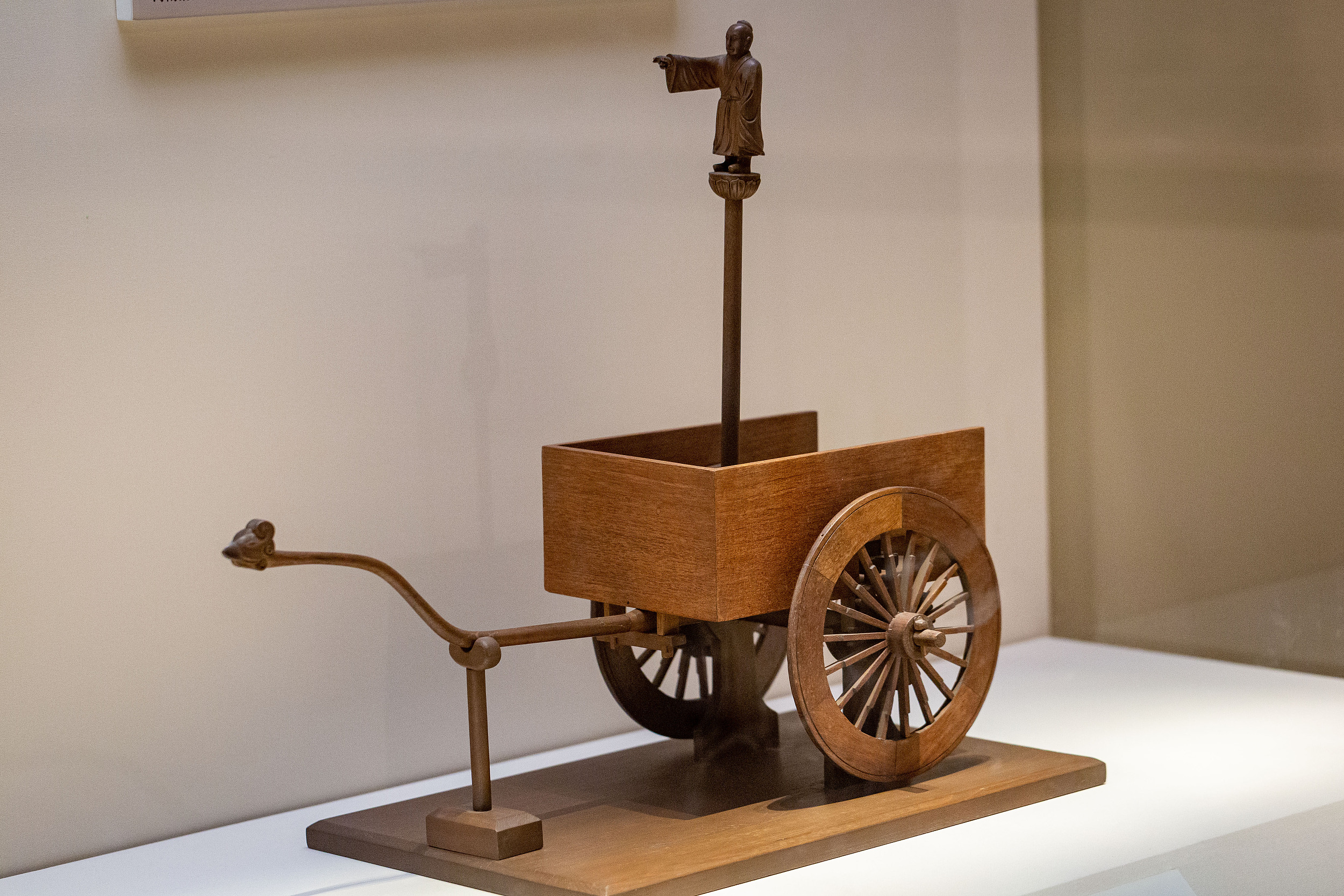This photograph features a detailed wooden cart, centrally positioned and box-shaped with an open back and two prominent wooden wheels on either side. The cart rests on a rectangular wooden plaque, secured by three wooden arms—two holding it firmly in place and one in the front supporting a protruding bar. Inside the cart, a long wooden pole extends outward, atop which stands a small figurine resembling a monk. This figure points outward with its right hand while standing on a round pedestal. The background reveals a white wall behind the cart and a yellow wall to its right, suggesting that the cart is displayed within an exhibition space, possibly an art museum. The cart's intricate design hints at it being a historical or cultural artifact, potentially inspired by ancient Chinese inventions. Reflections across the image indicate that it is housed within a display case, adding to its air of preservation and significance. The craftsmanship, possibly using cedar or pine wood, enhances its antique appearance, giving the impression it could be around a century old.